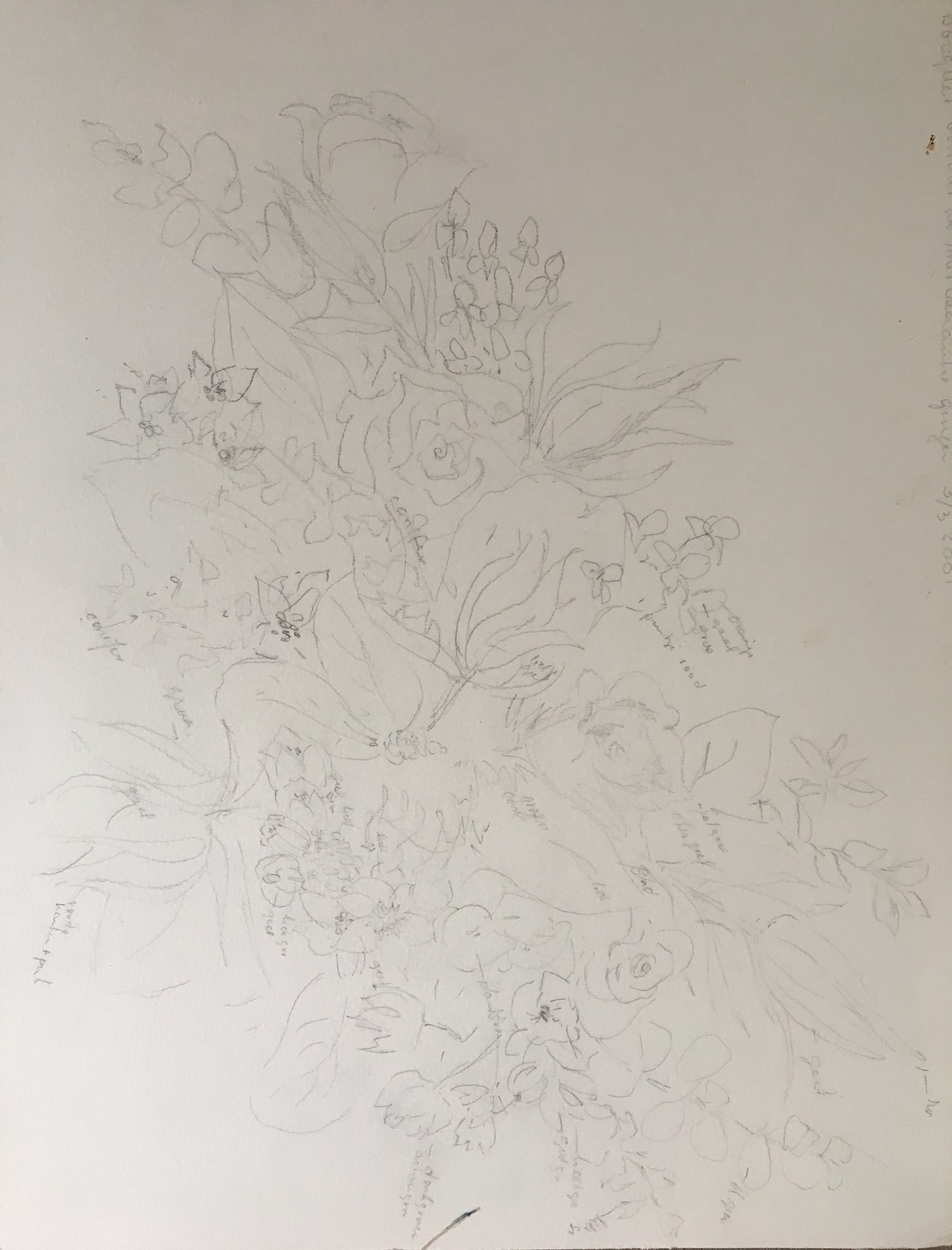This image is a vertical rectangular photograph or scan of a white piece of paper that features a lightly sketched bouquet of flowers. The drawing, done in regular dark lead pencil, stretches from the top left corner across to the bottom right, encompassing various floral designs. At the top left, there is an area dominated by leaves, alongside which might be a peony. As the sketch extends downward, it appears to include roses, some small three-petaled flowers or possibly baby's breath, and plant-like elements resembling ferns or fillers. In the right middle section, lilies can be seen, and more lilies are discernible at the center of the image. The bottom right corner includes additional roses and leaves. Across the entire sketch, lightly written and somewhat blurry pencil notes are scattered, though they are not legible. The paper itself appears white but has shadows in certain poorly lit areas, making parts of it look darker.